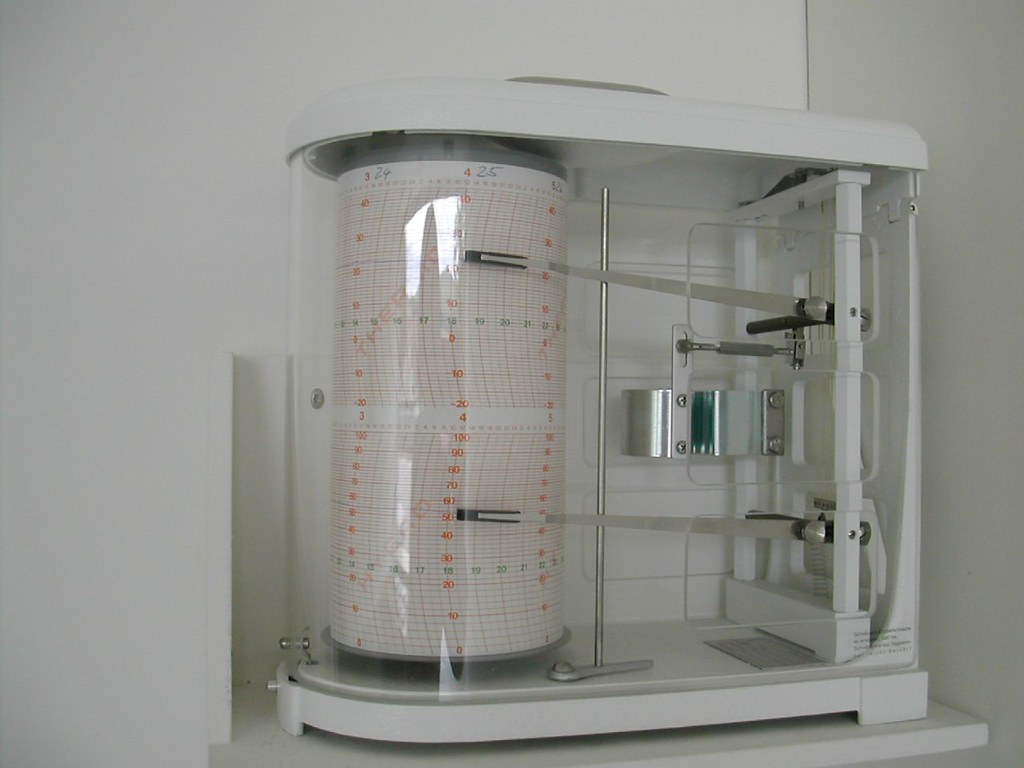The photograph captures an indoor scene with two white walls converging at a corner where a small white recessed shelf is mounted. Resting on the shelf is a compact instrument, appearing to be a seismograph, which is used for measuring earthquake activity. The device has a clear casing with a white base and contains two long rods that move vertically to draw lines on an attached spool of paper, which is adorned with various numerical markings. The casing of the seismograph features small, black lettering that is difficult to read, and the interior includes visible metal components and screws, indicating the machine's assembly.